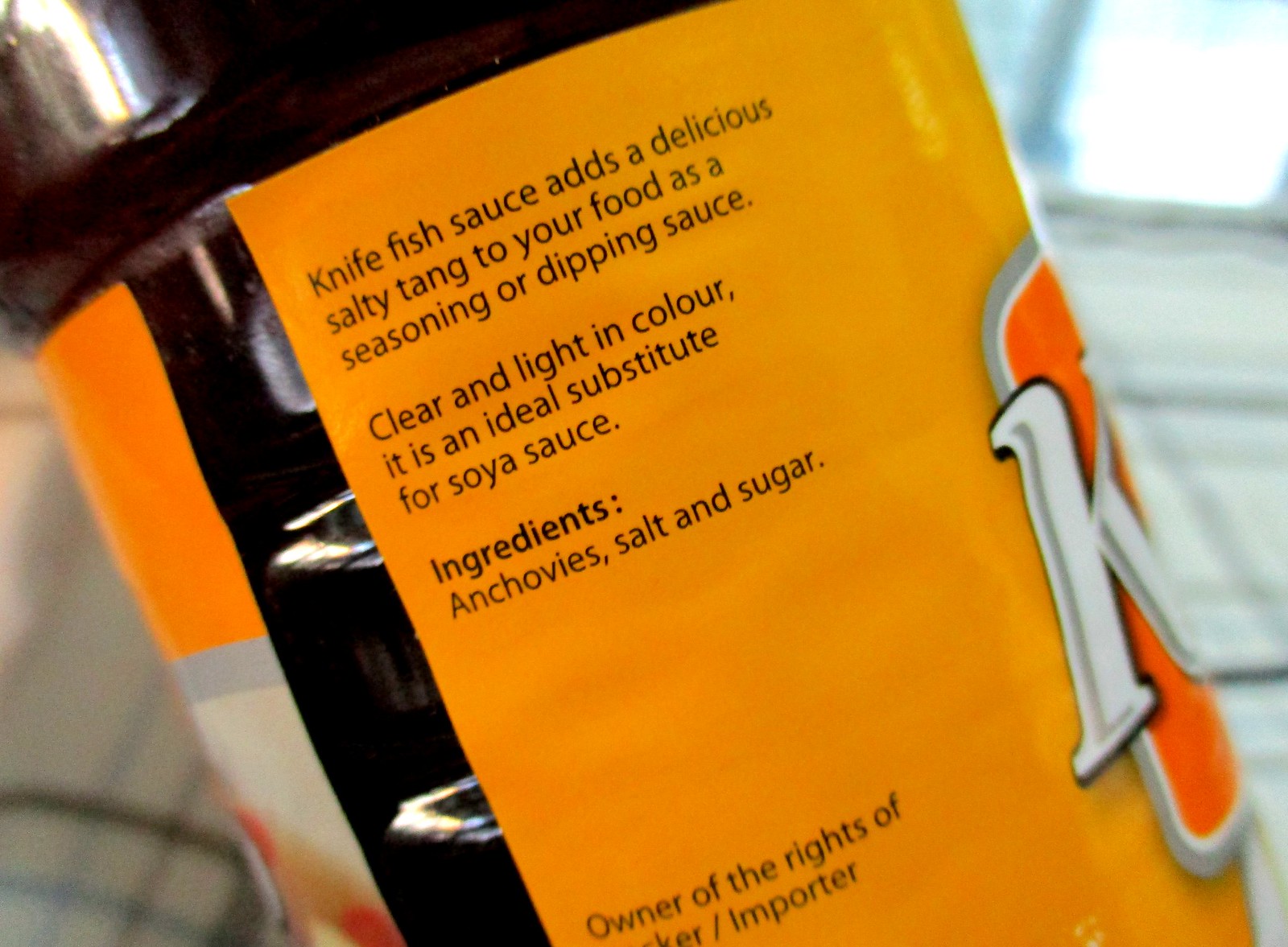The image features a close-up of a dark-colored bottle, which appears to be clear glass containing Knife Fish Sauce, as indicated by the partially visible label. The label, oriented diagonally approximately 45 degrees counterclockwise, is predominantly a yellowish-orange color with black text. The logo includes a large white "K" on an orange background, though the rest of the branding is not fully visible. The text on the label reads, "Knife Fish Sauce adds a delicious salty tang to your food as a seasoning or dipping sauce. Clear and light in color, it is an ideal substitute for soy sauce." The ingredients listed are anchovies, salt, and sugar. Additionally, at the bottom of the label, the text mentions "owner of the rights/importer," though some parts are cut out in the image.